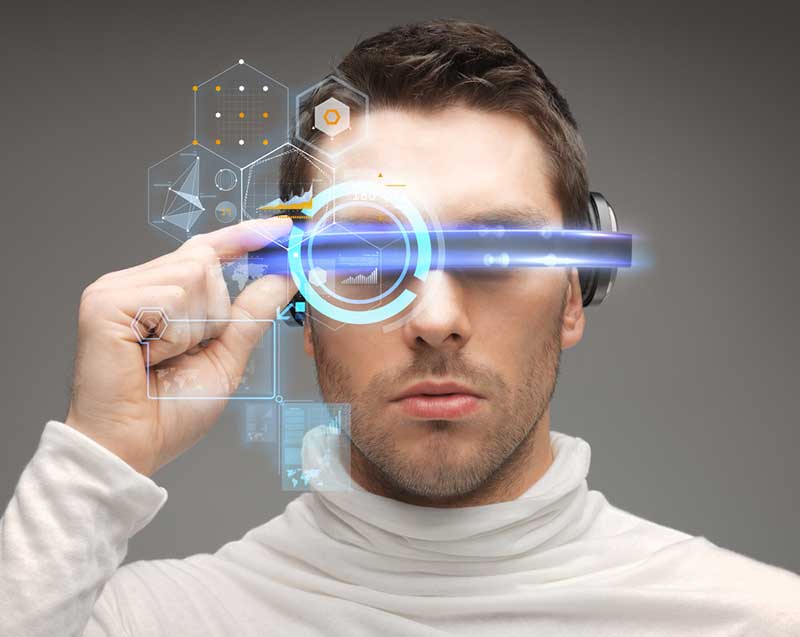The image features a close-up color photograph of a young man centered against a solid gray background. He has dark hair and a short stubble beard and is wearing a white turtleneck sweater with long sleeves that appears to have some folds, giving it a slightly textured look. The main focus is on the futuristic headgear he is wearing, which consists of a horizontal narrow band with glowing blue lights on the top and bottom borders and integrated speakers over his ears. He is adjusting this eye device with his right hand, pressing a button on the right side of his temple. Superimposed in front of him are intricate digital graphics, including circular highlights, hexagonal patterns, and various line art illustrations, indicating that he is interacting with some augmented reality interface. The digital images extend from his right eye, across his hand, down to his mouth, suggesting he is immersed in the virtual content projected through the device. The overall style of the image is a blend of photographic realism and line art illustration, likely serving as an advertisement for a high-tech, futuristic product.